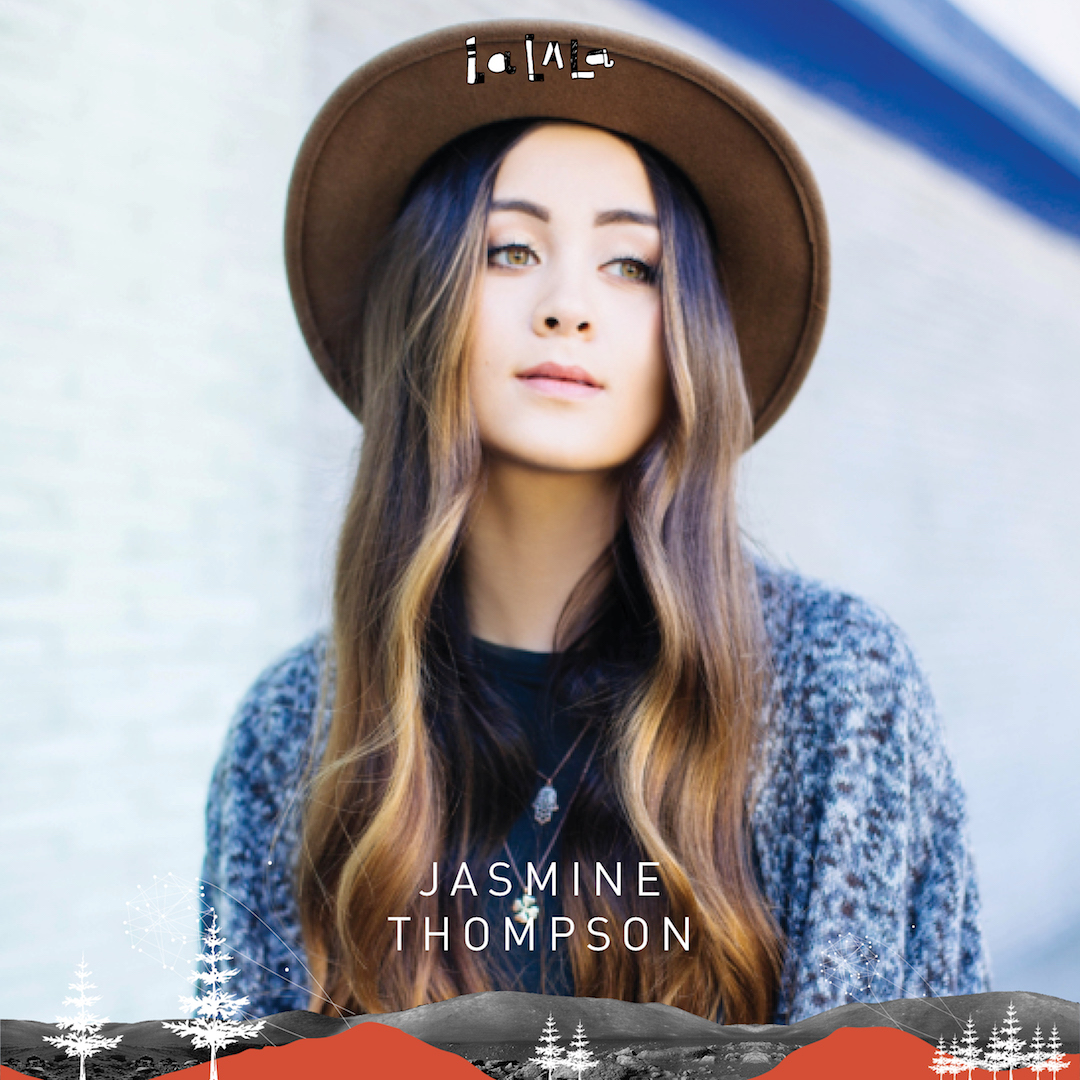The album cover features Jasmine Thompson, a woman with long, flowing hair cascading beneath a large fedora hat. She exudes an air of serene confidence in a stylish blue jacket, accented by a matching blue strap. The background is a pristine white, providing a stark contrast to the vivid imagery around her. Below Jasmine, light white trees and a blend of red, gray, and black mountains create a textured landscape, grounding the visual narrative. Above her, small symbolic illustrations add an element of intrigue. Jasmine Thompson's name is prominently displayed in elegant white lettering, neatly positioned to make a signature statement.